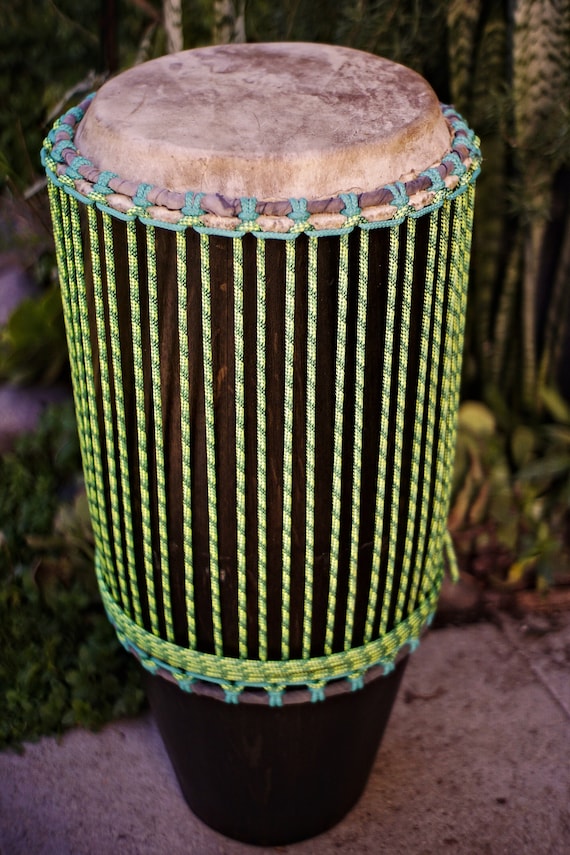This detailed photograph prominently features a unique musical drum, occupying almost the entire frame. Positioned outdoors on a concrete slab, the drum stands against a backdrop of slightly out-of-focus greenery. The drum top, crafted from a natural, leather-like material, exhibits a soft, beige tone marred by brown spots and scratch marks, perhaps from use. The cylindrical body of the drum is adorned with alternating bright green and dark green nylon ropes, running vertically halfway down before wrapping around the drum horizontally in a band, creating a striking parrot green paracord aesthetic. Despite its tall and colorful appearance, the drum’s base subtly resembles the shape of a flower pot. The composition is highly zoomed in, directing full attention to the drum’s intricate texture and vibrant details.